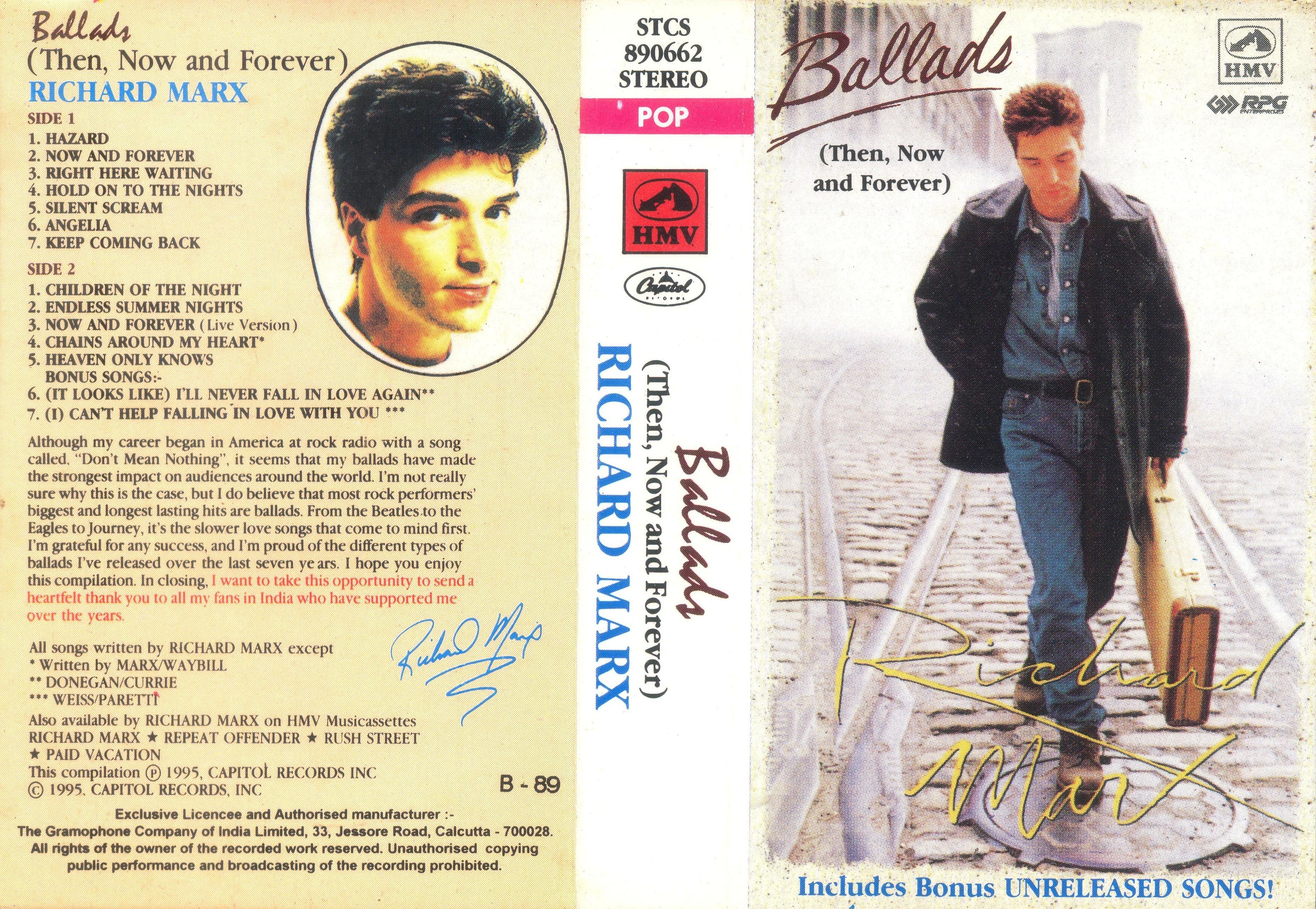The image is a vintage music cover for Richard Marx's collection of songs titled "Ballads: Then, Now, and Forever." The cover is divided into two sections. On the right, against a foggy city backdrop, Richard Marx is walking on concrete streets. He is a white man with short brown hair, dressed in a black leather jacket, a blue jean button-up shirt over a t-shirt, jeans, and brown shoes. He carries a light brown guitar case in his left hand, his right hand tucked into his jacket pocket. The title "Ballads" appears in cursive, followed by "(Then, Now, and Forever)" underneath. Below this, "Richard Marx" is written in gold.

On the left side, the cover features a tracklist for sides one and two. Side one includes songs like "Hazard," "Now and Forever," "Right Here Waiting," "Hold On to the Nights," "Silent Scream," "Angelia," and "Keep Coming Back." Side two features another set of seven songs. Additionally, this side includes a close-up of Richard Marx's face encircled in black, his signature in yellow, and various details such as the serial number "STCS 890662," the labels "STEREO" and "POP," and the HMV logo with a red box and oval image. The cover mentions "Includes Bonus Unreleased Songs" in capital letters with an exclamation point. There's also a descriptive section about the artist and the recording, including stamps, numbers, and more signatures. Overall, the cover evokes a nostalgic feel, reminiscent of old-school cassette inserts.